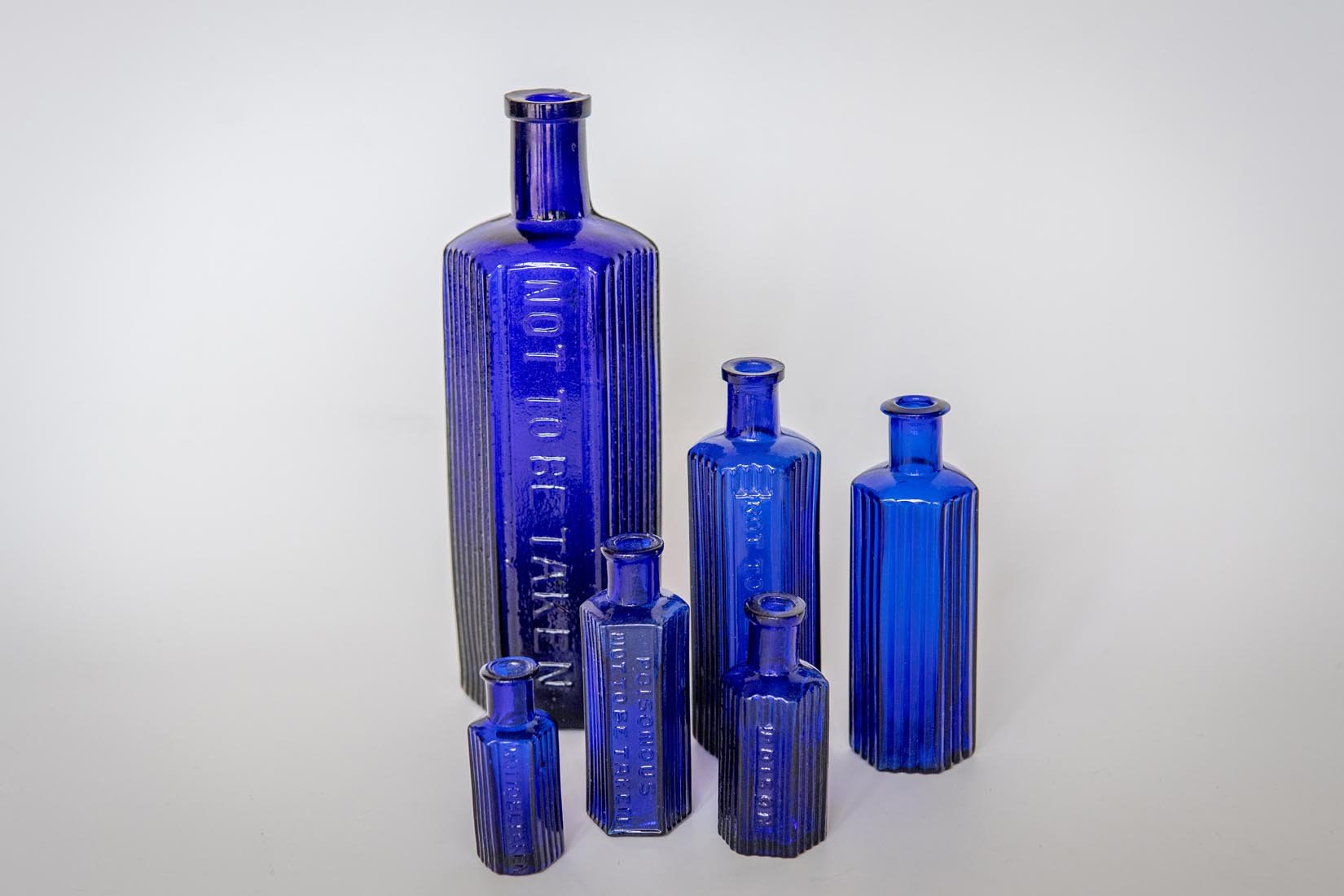The monochrome photograph, set against a soft, plain grey background, features six antique glass bottles meticulously aligned. Each bottle shares the same vintage design, characterized by intricate indented lines along their sides and a flattened front surface. These bottles vary in size, ranging from a modest miniature, akin to complimentary hotel provisions, to a substantially larger one. The most prominent bottle, along with at least a few others, bears a clear vertical inscription reading "NOT TO BE TAKEN," suggesting they were once used for medicine or hazardous substances. Despite their old-fashioned shape and absence of corks, the bottles exhibit a distinct blue hue, unifying them as a cohesive collection.